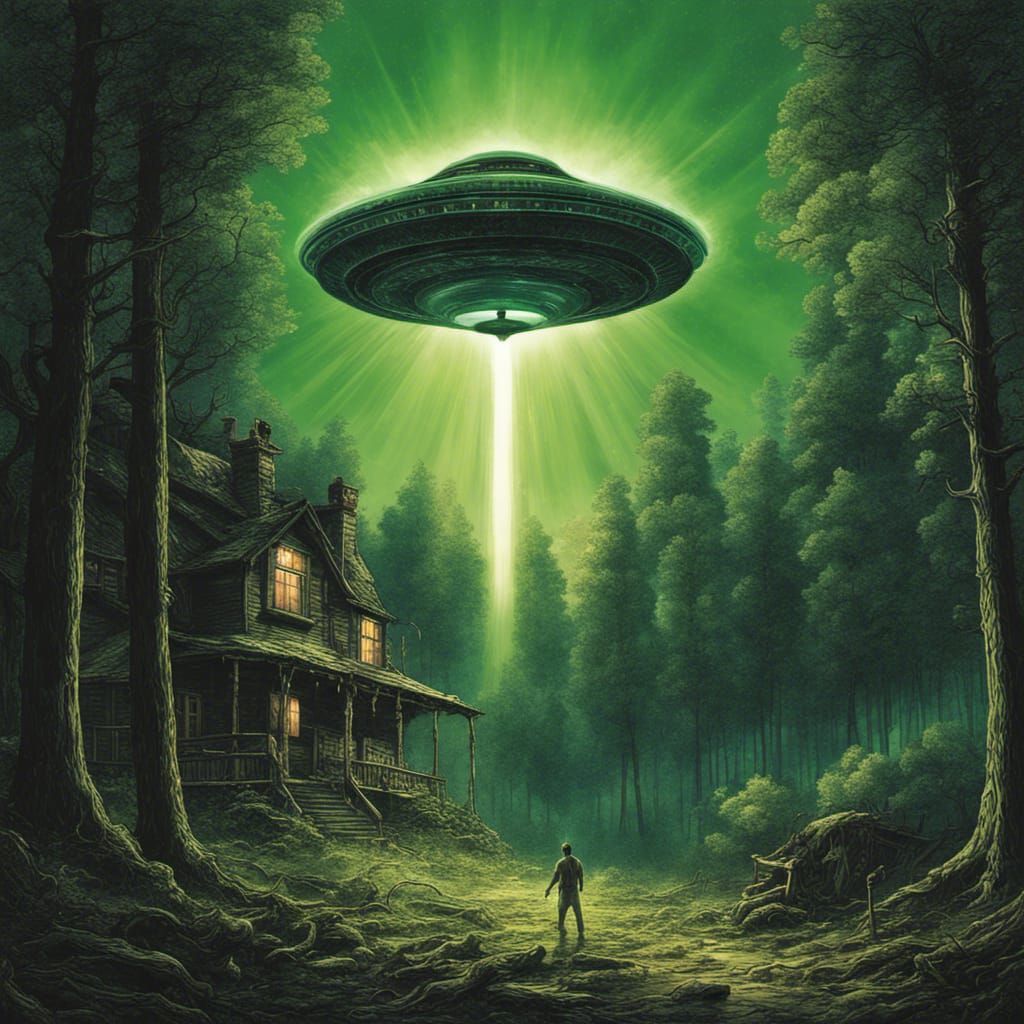The image illustrates an eerie, AI-generated forest scene under a green, starry night sky. Dominating the landscape is a glowing, disc-shaped UFO hovering above and to the right of a two-story wooden log house, complete with a porch and glowing yellow windows, implied to be inhabited. Trees, mostly cedar and evergreen, surround the house, framing a clearing with a man standing in the foreground. A striking green and white laser beam extends from the UFO towards the man. The earthy brown dirt contrasts with the predominantly green and yellow hues, accentuating the overall ominous and surreal ambiance. The forest floor shows odd visual artifacts, particularly around the tree roots and ground, hinting at the AI-generated nature of the artwork.